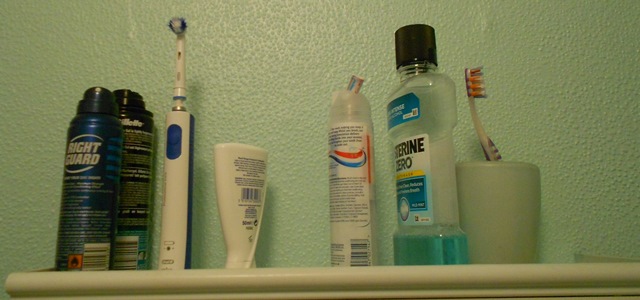A photograph of a white bathroom shelf against a light seafoam green, textured wall, featuring various hygiene products. On the left side of the shelf, there's a blue can of Right Guard deodorant, followed by a partially obscured black container. Next, there is a worn blue and white electric toothbrush beside a red, white, and blue container which could be either Aquafresh toothpaste or shaving cream. Further along, the shelf holds a bottle of Listerine mouthwash and Listerine Zero. On the far right, a cup containing an orange and purple toothbrush completes the arrangement. The background wall displays a unique, slightly bubbly or knockdown paint texture that enhances the overall appearance of the bathroom setting.